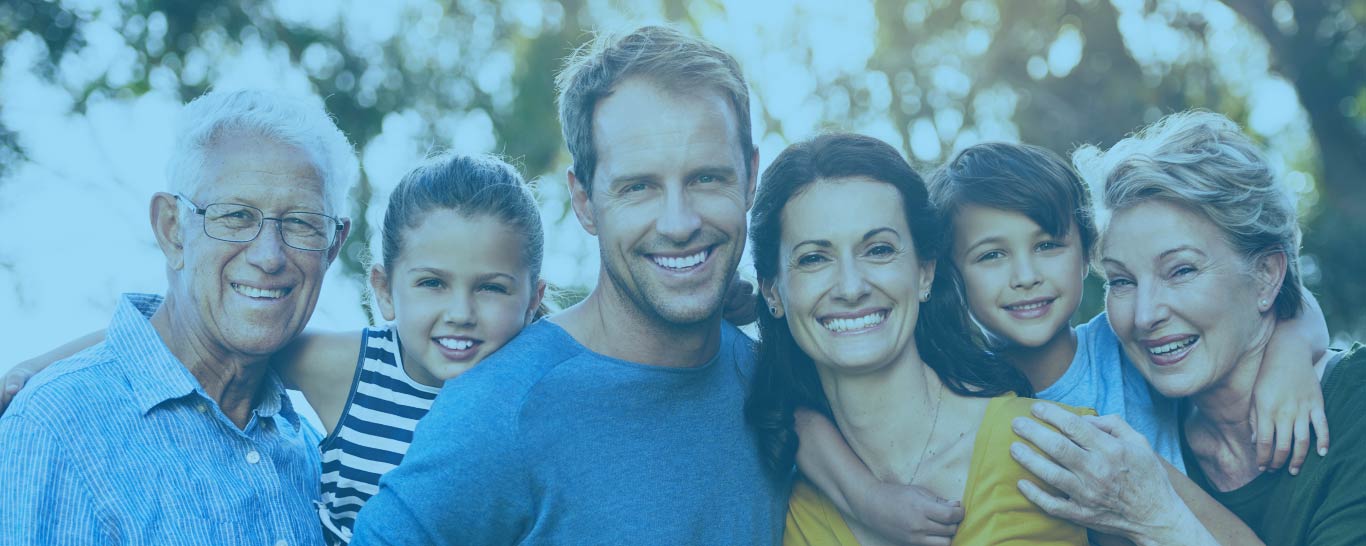This is a detailed panoramic image that appears to be a posed depiction of a multi-generational Caucasian family, possibly for a commercial or stock photo. From left to right, the photograph features:

- An older man with white hair and glasses, smiling at the camera. He is wearing a blue and white striped button-down collared shirt. He seems to be the grandfather.
- Next to him is a young girl with brown hair pulled back. She is smiling at the camera and is dressed in a blue, navy blue, and white tank top.
- In the center, a middle-aged man, who appears to be the father, is smiling at the camera. He has light brown hair, a slight stubble, and is wearing a blue t-shirt or sweater.
- Beside him is a woman with brown hair also pulled back, smiling at the camera. She is wearing a yellowish v-neck shirt and has a small boy with brown hair in a light blue shirt wrapped around her neck.
- Finally, to the right of the boy is an older woman, likely the grandmother, with short gray hair and a green shirt.

All the family members are closely bunched together, creating a harmonious and smiling tableau that has a slight blue haze to it, giving a uniform hue to the image.